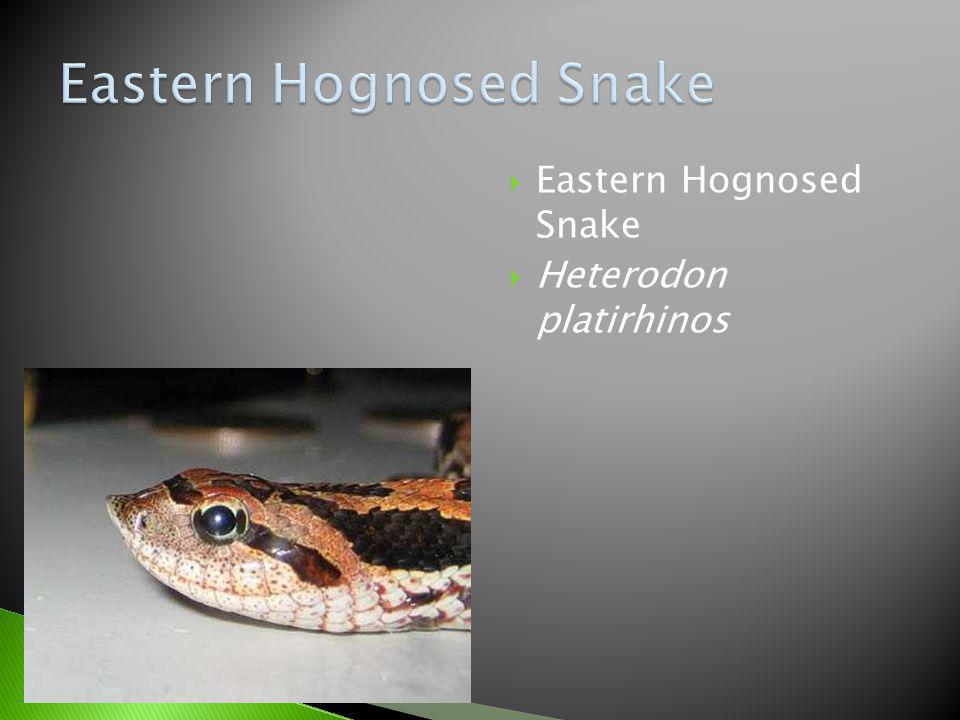The rectangular image, likely from a textbook or informational sign about reptiles, features the Eastern Hognose Snake. The title "Eastern Hognose Snake" appears in light blue text at the top, in either Papyrus or Comic Sans font, with each word's initial letter capitalized. The background transitions from darker, almost black, tones in the upper left and lower right corners to a lighter gray towards the center, creating a gradient effect. 

In the bottom left corner, there is a triangular green and black design element. Just above this design sits a horizontally aligned photograph of the Eastern Hognose Snake. The photo showcases the snake's head, facing left, with detailed coloration: a tannish face, brown stripe descending from its eye, a tan stripe above that, and a black stripe even higher. The snake's belly is white with a few black markings. The surface beneath the snake appears smooth and pale blue, with what looks like coins in the background.

On the top right of the image, two green bullet points are listed vertically. The first bullet point reads "Eastern Hognose Snake" in white text, with the words capitalized similarly to the title. Beneath it, in italicized white text, is the snake's scientific name, "Heterodon platyrhinos."

Overall, the image combines a detailed photograph with textual information, providing a comprehensive visual and written description of the Eastern Hognose Snake.